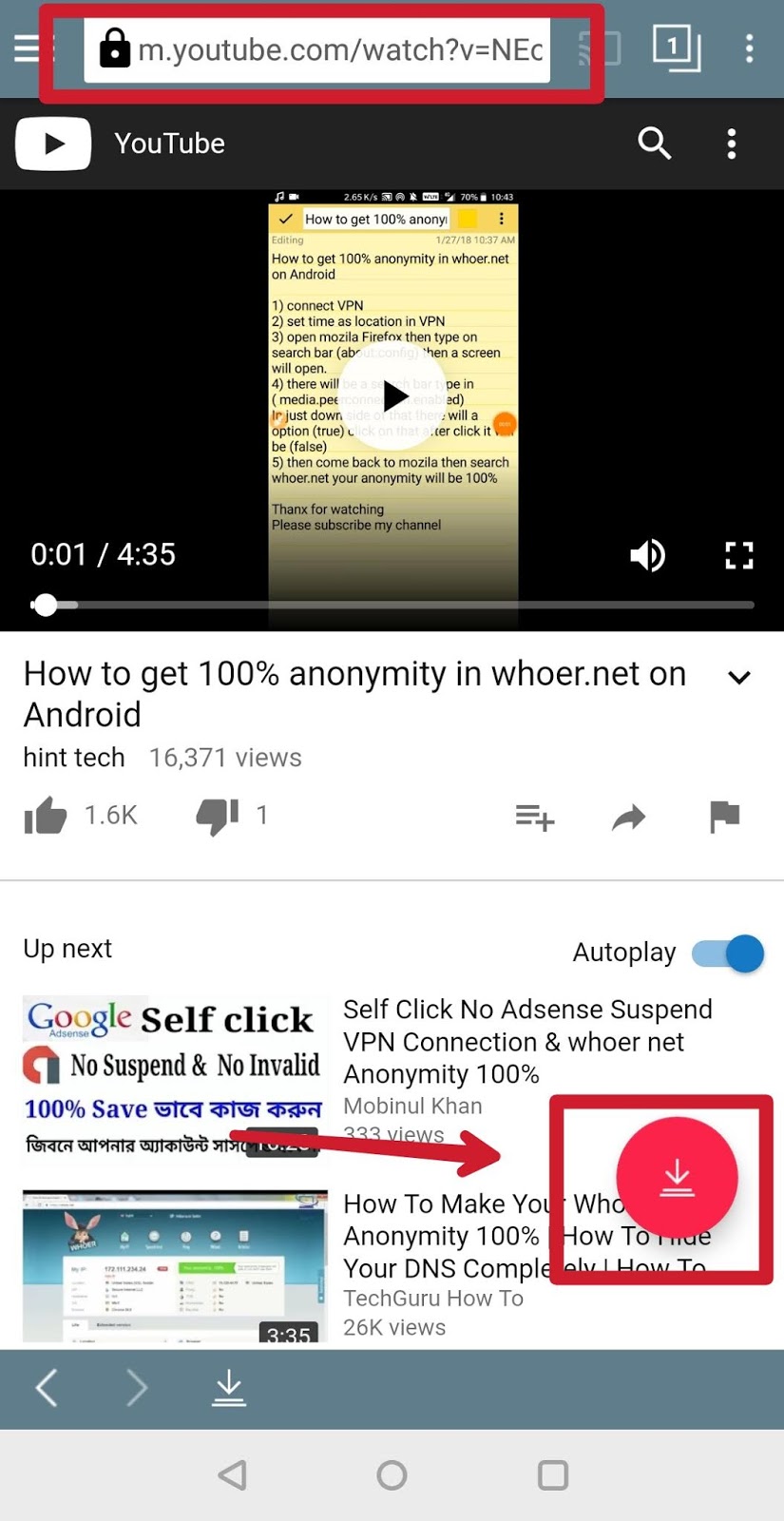This vertically-oriented image, likely captured from a smartphone, features a screenshot of a YouTube video paused at the one-second mark. The top part of the screen displays a slate gray navigation bar with three horizontal white lines in the upper left-hand corner, indicating a menu. To the right of the menu icon is a search bar with a padlock icon, emphasized by a thick red outline. On the upper right, there are icons: a box with a number "1" inside, another partial box behind it, and three vertical dots for more options.

Beneath this, a gray and black background prominently shows the YouTube play button, a magnifying glass, and more options circles. The current video paused is titled "How to Get 100% Anonymity," and it appears to be from a channel named "Hint Text." As indicated, the video has 16,371 views, 1.6 thousand likes, one dislike, and various options for interaction.

Further detailing includes a progress bar showing 1 second out of a 4-minute and 35-second video. Below the video, the "Up Next" section lists a video titled "Google Self Click: No Suspend and No Invalid" with additional descriptions. There is a red arrow pointing to a specific part of the text featuring a red box and a circular icon with a downward-pointing arrow for emphasis. The background of the entire screenshot uses the white from the computer screen, giving it a clean and uncluttered look.